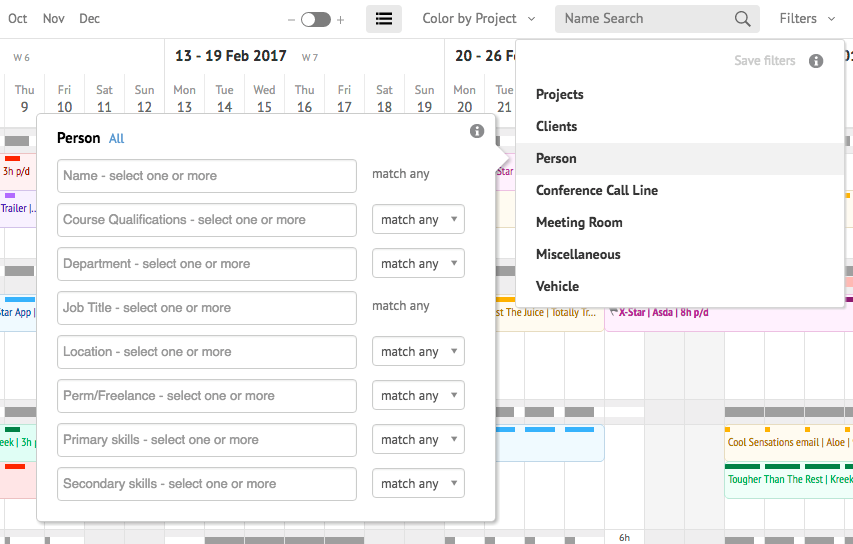The image showcases a detailed electronic calendar interface with organizational tools and filters. At the top of the interface, the months "October," "November," and "December" are displayed, accompanied by a plus and minus toggle switch, currently set to the minus position. A square button with three clickable lines shows a drop-down menu labeled "Color by Project." Adjacent to this is a search bar with a magnifying glass icon and a filters button with another drop-down menu.

The interface includes several opened boxes over the vibrant calendar, each categorized under different headings such as "Projects," "Clients," "Persons," "Conference Call," "Meeting Room," "Miscellaneous," and "Vehicle." The "Persons" category is expanded, revealing links like "All," "Name," "Course Qualifications," "Department," "Job Title," "Location," "Perm," "Freelance," "Primary Skills," and "Secondary Skills."

The background calendar is a mosaic of colors, including shades of purple, yellow, green, blue, and red, highlighting different scheduled activities. A specific week, from February 13th to February 19th, 2017, is distinctly marked, indicating a detailed, well-structured view for that period.